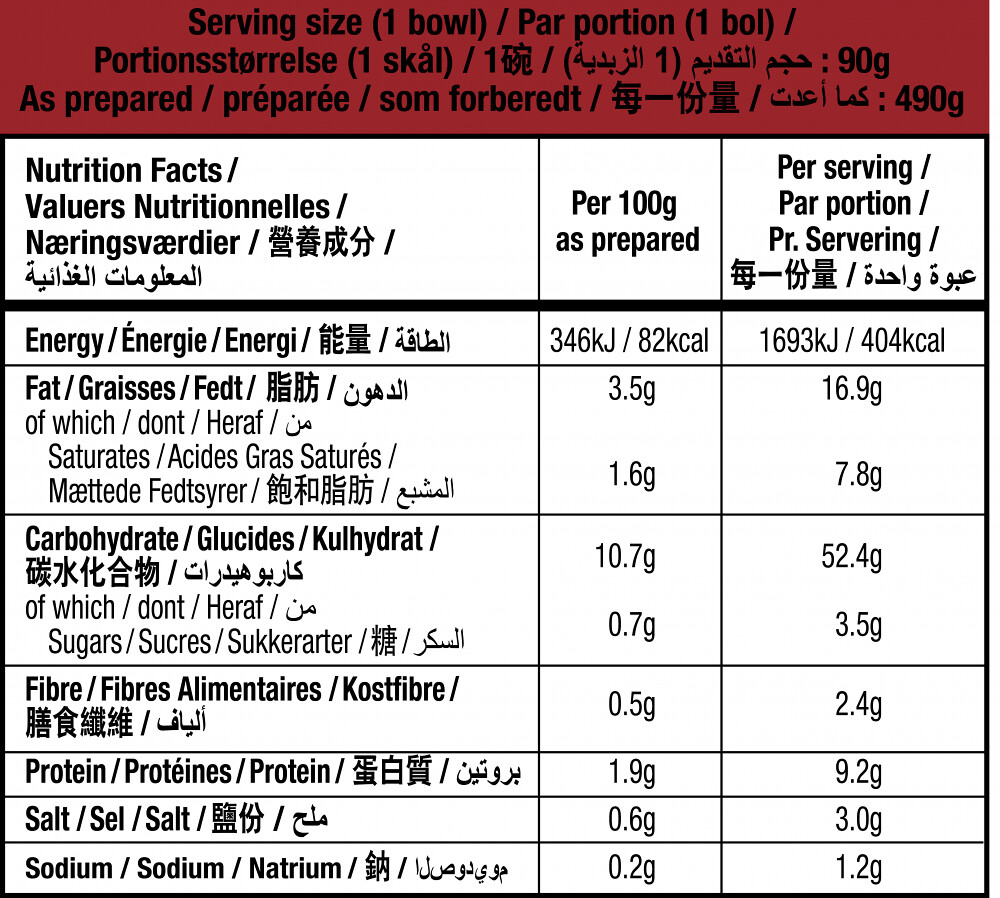This color image showcases a detailed nutrition label from a food product. The top portion of the label features a red background with bold black font stating "Serving size: one bowl." Directly underneath, the label indicates "As prepared: 490 grams" and includes additional text in what appears to be Thai characters. Below this section, a white background with black text provides the nutrition facts, detailed as "per 100 grams as prepared" and "per serving." Energy content is listed as 346 kilojoules (82 kilocalories). It also includes information on carbohydrates, fiber, protein (1.9 grams), fat (3.5 grams), salt, and sodium levels. The label is multilingual, with text in English and several other languages, possibly including Arabic.